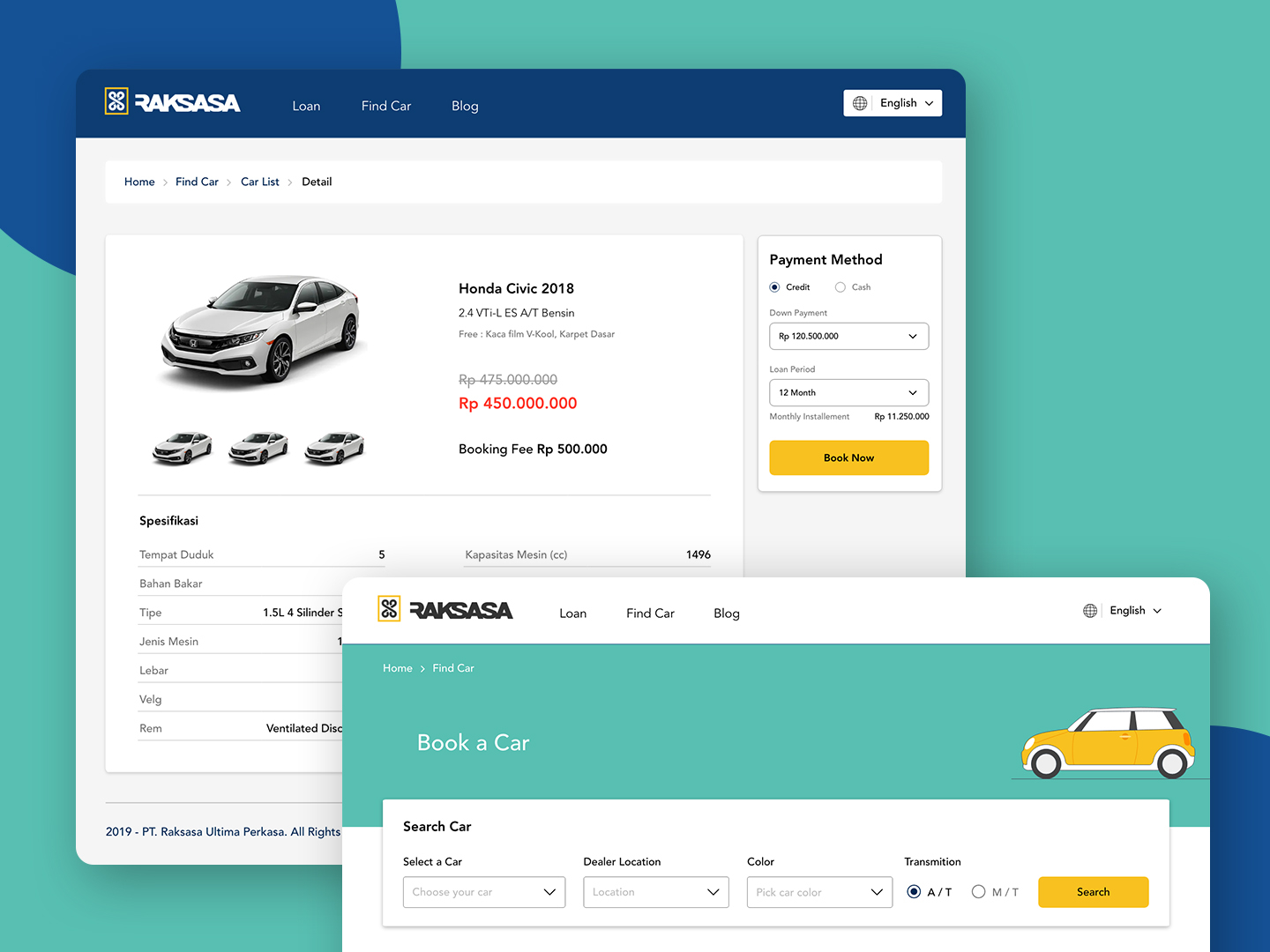The image showcases a webpage from a company named "Rack Sasa," which appears to be an automotive business. The top section of the page features a blue strip displaying the text "First Car," along with options for "Loans" and "Blog." Below that, there is a light gray box with white interior containing a navigation menu with options labeled "Home," "Fixed Car," "Car Use," and "Detail."

Central to the image is a photograph of a white 2018 Honda Civic 2.4 ES. Beneath the car's image, there are three different style options displayed. The car is priced at RP 450,000,000, marked down from its original price of RP 475,000,000. Some notable features of the car are listed as well.

On the right side of the webpage, a section describes the available payment methods, which include cash and credit, with a field for inputting payment information. Additionally, there is a pop-up window from the same company titled "Book a Car," which allows users to select a car, specify a dealer location, choose a color, and perform a search.